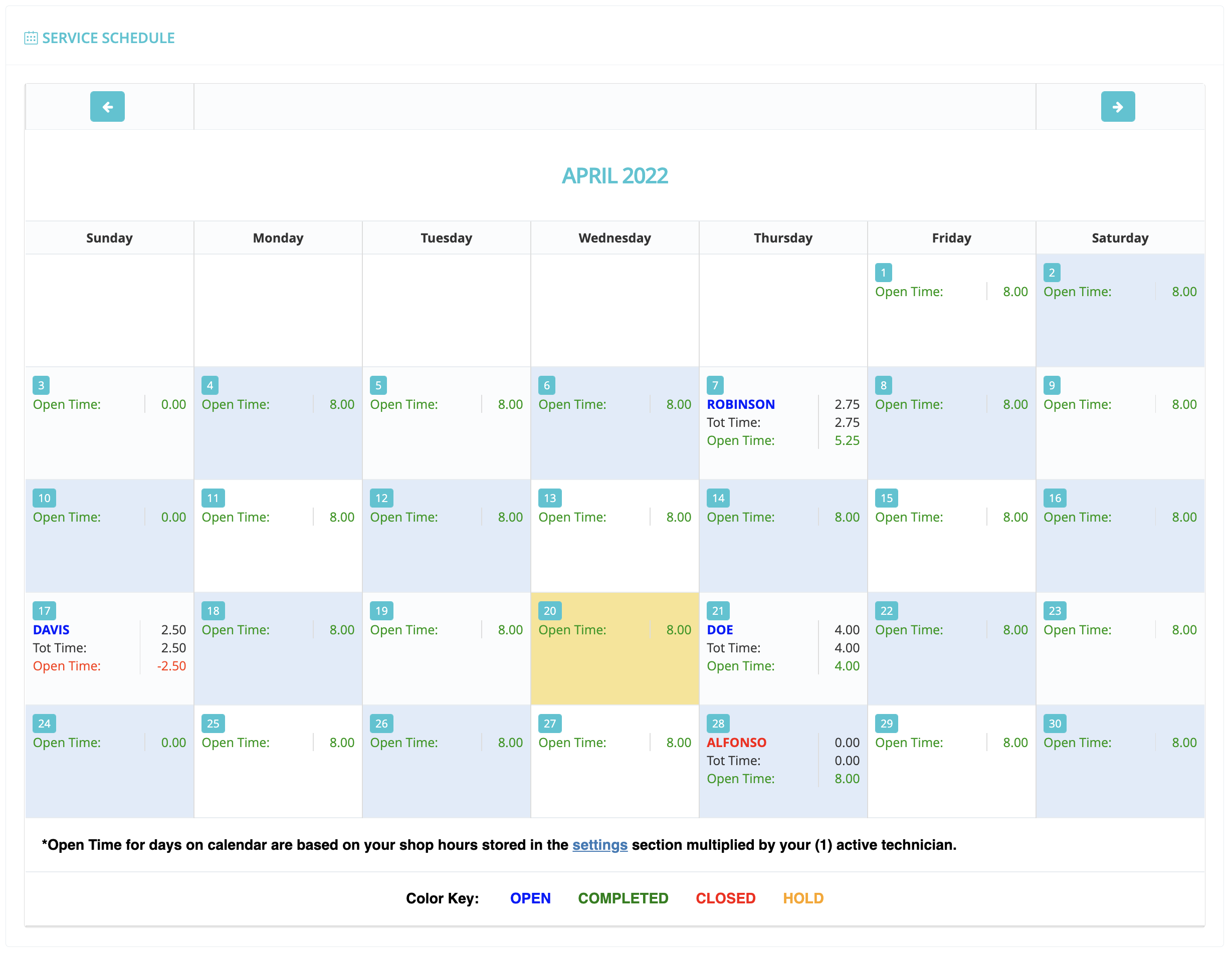The image is of a detailed service schedule calendar for the month of April. In the top left corner, it is clearly marked as a "Service Schedule." To the left below this title, a white left-pointing arrow is displayed inside a blue section. Conversely, in the top right corner, a similar blue section houses a right-pointing arrow. 

The calendar grid is laid out with days of the week—Sunday through Saturday—written in black across the top. The date blocks, where each day starts, are marked with a blue background and white numeric labels. April begins on a Friday, denoted as the 1st, and ends on a Saturday, the 30th.

Each date block includes an "Open Time," generally listed as 8:00 AM, except for Sundays where the open time is often recorded as 0, indicating no service. However, an exception appears on the 12th, which includes additional notes: "Davis" with a total service time of two and a half hours, entirely during open hours.

Highlighting for specific purposes includes one notable day: the 20th of the month. This block is completely colored in orange with text in green, indicating a special status according to the calendar's key.

At the bottom, a color key provides important context for interpreting the calendar: blue denotes "open," green signifies "completed," red means "closed," and orange indicates a "hold" status. 

In essence, this calendar meticulously tracks service scheduling details, including specific times and statuses for each day of April.